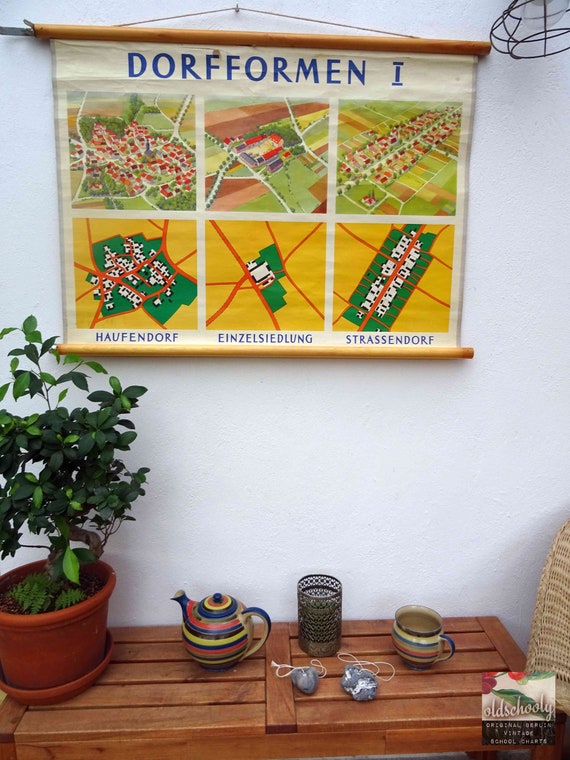In a cozy room with a whitish-gray wall, a wooden shelf at the bottom displays an assortment of items, creating a charming vignette. The shelf holds a green-leaved plant in an orangey-brown pot, a multicolored ceramic teapot, a filigree candle holder, a coffee mug, and two small ornaments with strings attached. A label on the shelf reads "Old Skoolie, Original Berlin Vintage School Charts." Above the shelf, a fabric banner hangs from a nail, supported by bamboo rods at the top and bottom. The banner, inscribed with "Dorf Formen 1" in blue letters, features six square illustrations, arranged in two rows of three, depicting various towns. Each pair of images showcases different views, labeled as Hofendorf, Einzel-Siedlung, and Strassendorf. The illustrations, segmented into different maps with hues of yellow, green, and orange roads, offer a detailed, vintage feel to the room.